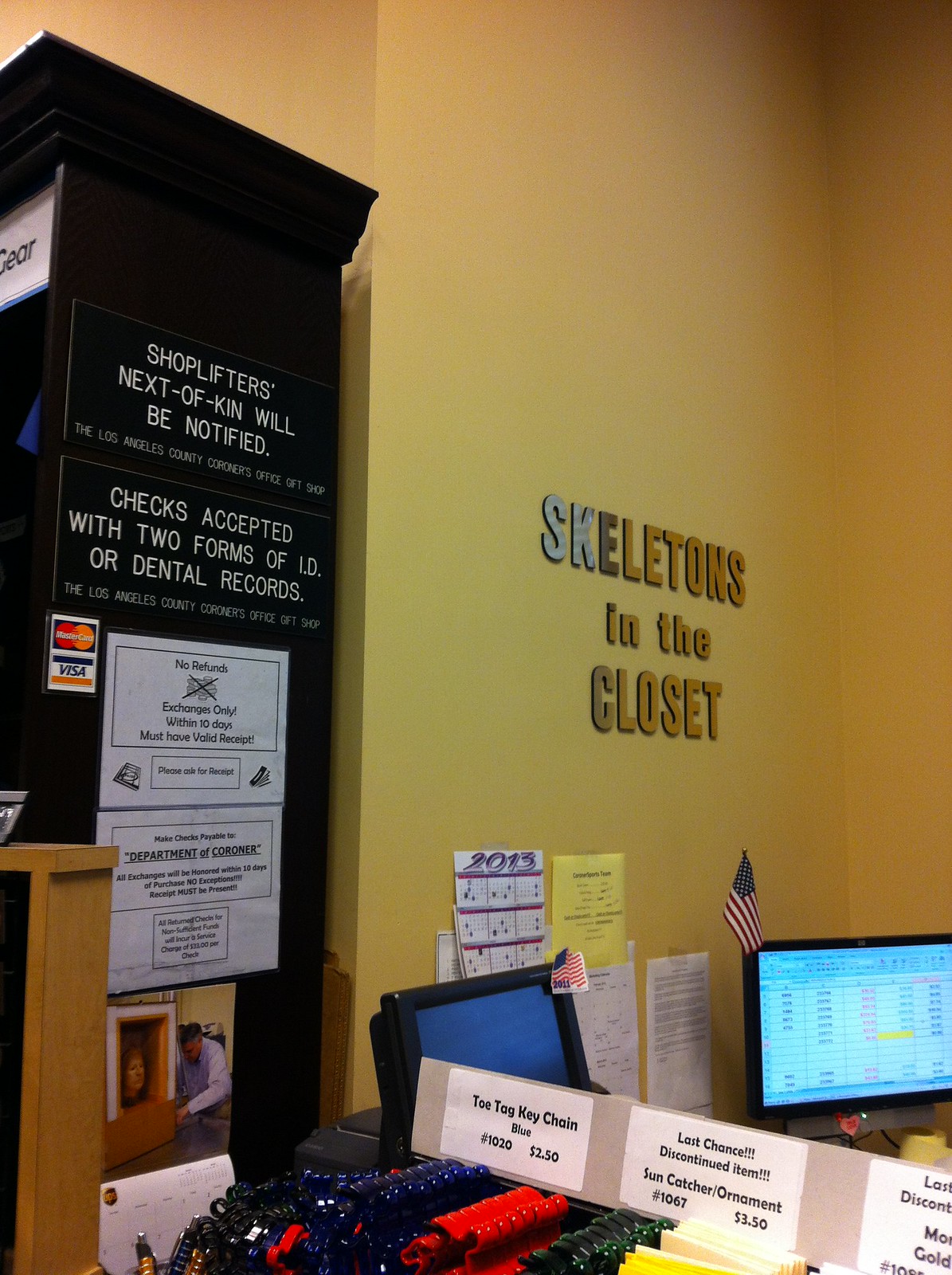In the image, the background wall is painted in a yellowish tone, prominently displaying a phrase in large letters: "SKELETONS IN THE CLOSET." The words "SKELETONS" and "CLOSET" are in all caps, with the letters S, K, and E in "SKELETONS" highlighted in a different shade, featuring bluish and white speckles while the E is slightly darker. To the left, on a black cabinet, there is a detailed sign stating, "Shoplifters next of kin will be notified. The Los Angeles County Coroner's Office Gift Shop. Checks accepted with two forms of ID or dental records. MasterCard and Visa accepted. No refunds; exchanges only within 10 days with a valid receipt. All exchanges will be honored within 10 days of purchase, no exceptions. Returned checks or non-sufficient funds will incur a $33 service charge." Below this, a calendar featuring a UPS symbol is visible. To the right, beneath the "SKELETONS IN THE CLOSET" phrase, there is a 2013 calendar and some unreadable papers taped to the wall. Below this setup, a closer look reveals an array of items for sale: T-tag keychains in blue (number 1020, priced at $2.50), and a "last chance" discontinued item, a sun catcher ornament (number 1067, priced at $3.50). The assortment also includes keychains in blue, red, and green. In the foreground, two computer monitors are decorated with American flags, and one monitor displays the year 2011. The scene highlights a quirky gift shop atmosphere with a morbid sense of humor, emphasizing details down to the transaction policies and itemized goods.